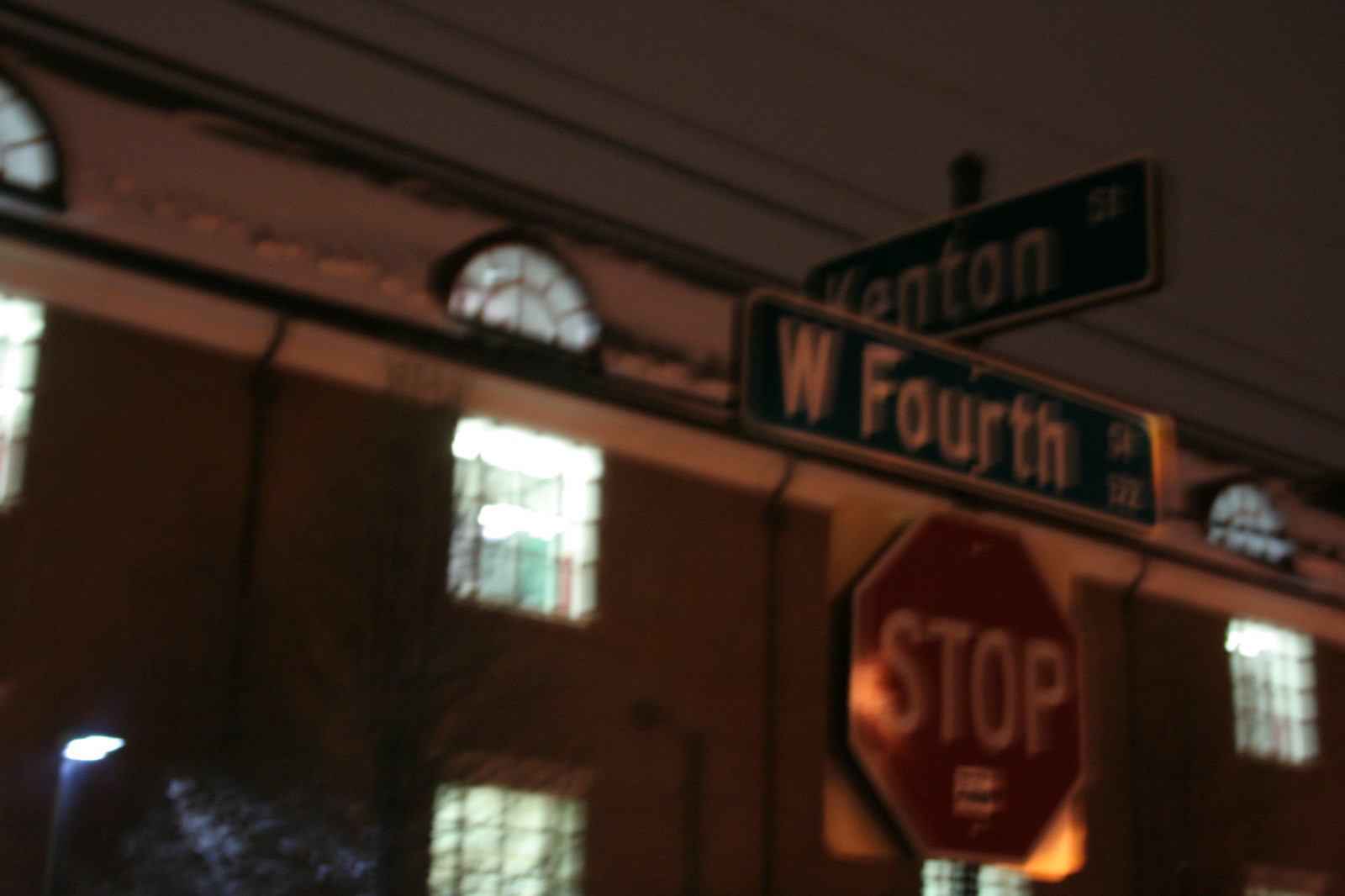In this image, a series of street signs are prominently displayed, though slightly blurred due to the image's lower resolution. At the top, the sign reads "Kenton Street," while just below it, another sign designates "W 4th Street." The latter also has an illegible string of numbers in the bottom right corner. Positioned directly beneath these street signs is a large, clear red stop sign. In the background, a substantial building can be seen with multiple floors and numerous windows illuminated by white lights, suggesting activity within. Above the scene, the sky appears overcast, casting a gray and gloomy atmosphere over the setting.